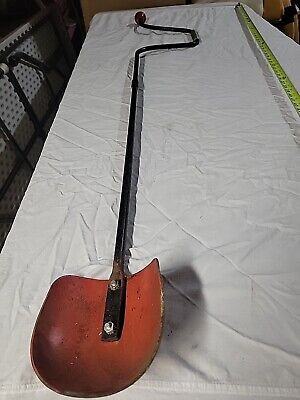The image depicts a long, slender tool resting on a white rectangular table covered with a white, wrinkled tablecloth that features green and gray stripes. The table appears to be part of a work area, possibly in a room with wrought iron chairs visible in the background. The tool resembles a shovel but has distinctive features, such as a scoop or spade that looks brown or red, a handle made from a black metal rod that extends approximately four feet, and a silver bolted joint. The handle deviates near the top to form a U-shaped piece of metal, which is unusual for a typical shovel. Additionally, there is a hand crank attached to the end of the rod, suggesting it might also function as some sort of stirrer, potentially for use on a boat, though its exact purpose remains unclear. To the right of the tool, a yellow tape measure is visible, indicating that measurements are being taken, with some marks suggesting the tool could be as long as six feet. On the left side of the table, there's a folded-up table leaning against the wall.